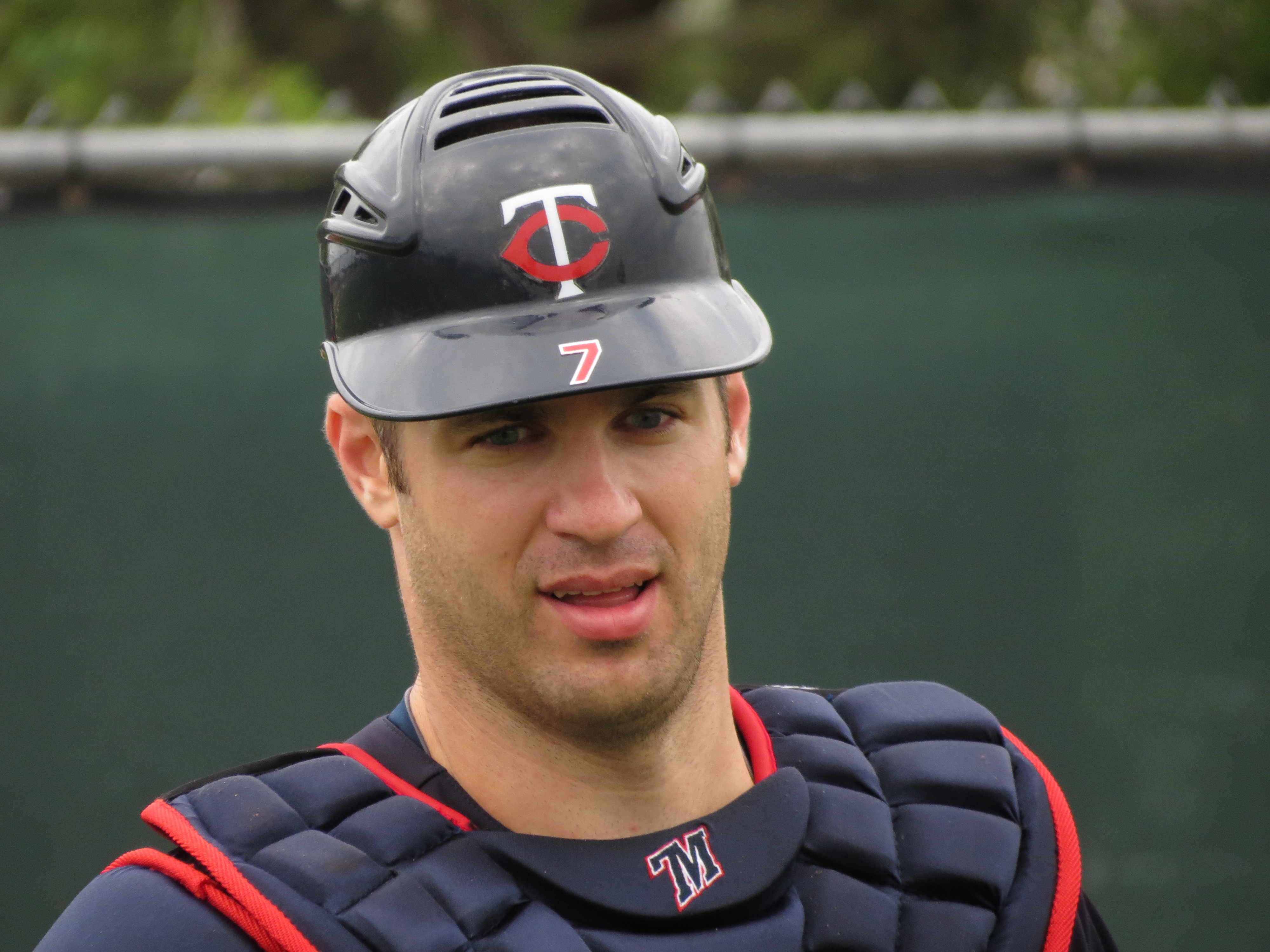The image depicts a baseball player, specifically a catcher, shown from the neck upwards. He is wearing a protective, padded chest guard that is navy blue with red trim and has a rubbery appearance. The helmet, also navy blue with red detailing, bears the number 7 and the initials "TC." Visible in the background are green fields, a gray wall, and some trees. There is minimal view of his uniform, emphasizing the protective gear and helmet.